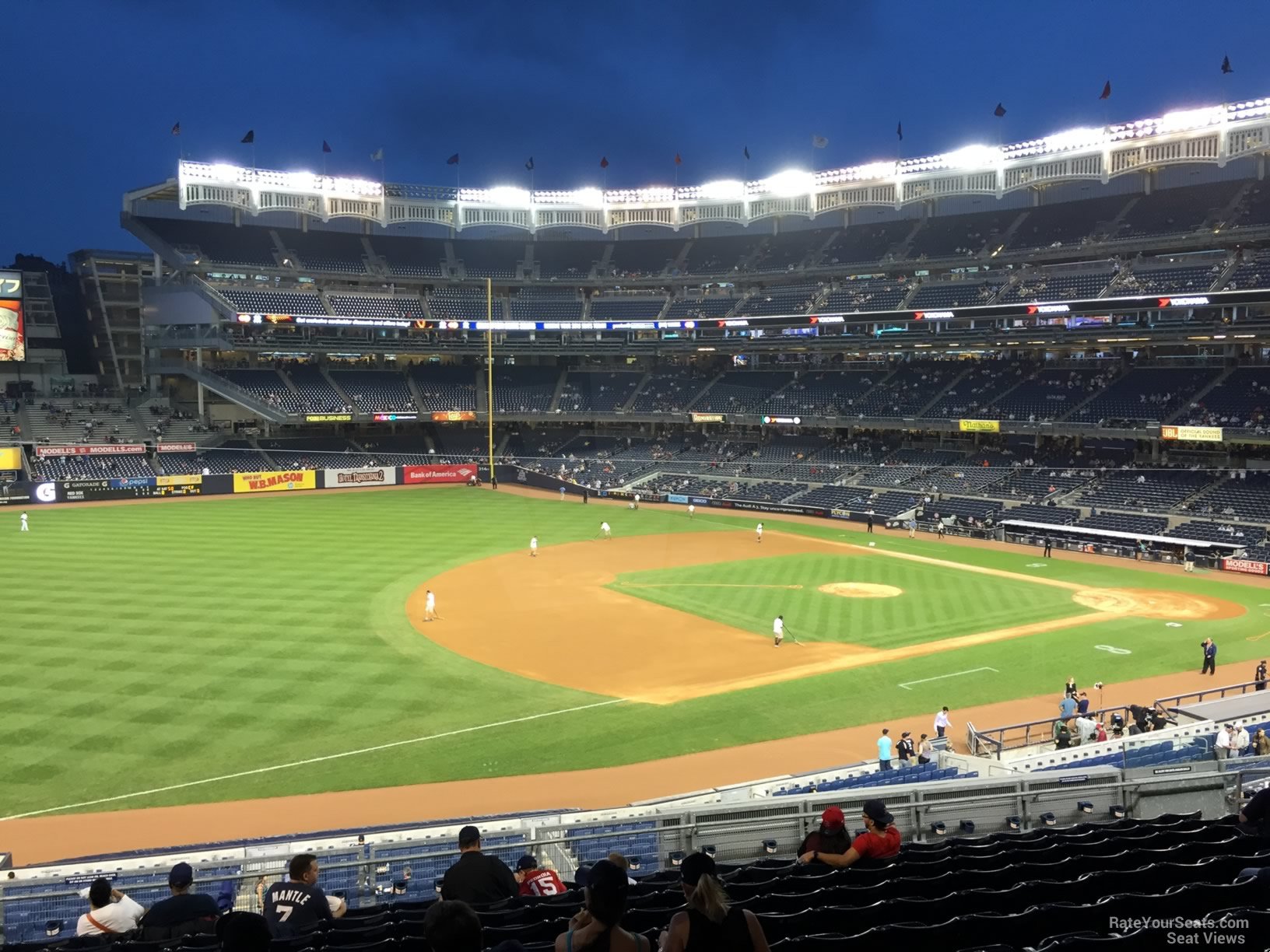This detailed color photograph, taken near sunset, captures an interior view of Yankee Stadium. The sky above is a dark blue, illuminated by the bright floodlights perched atop the stadium's structure. The image, oriented in landscape format, shows the field from a lower section of the stands, behind third base, angled towards the outfield. 

The green playing field is meticulously maintained, featuring a checkerboard pattern created either by mowing or artificial turf. The dirt areas around home plate, the pitchers mound, and the bases are well-tended, possibly by groundskeepers visible in the image. 

Distinct levels of stadium seating fan out around the field, with multiple flags flapping at the top. While the stands are not filled to capacity, various fans are spread out in the lower and upper sections, indicating the game may just be beginning or a practice session is underway. Security staff are positioned along the dirt track encircling the bases. 

Players in white uniforms are scattered across the field, although no batting activity is currently happening. The backdrop features sponsor advertisements and colorful banners along the fence. The photograph also includes a credit in the bottom right corner: “RateYourSeats.com seat views,” emphasizing its representational realism style.